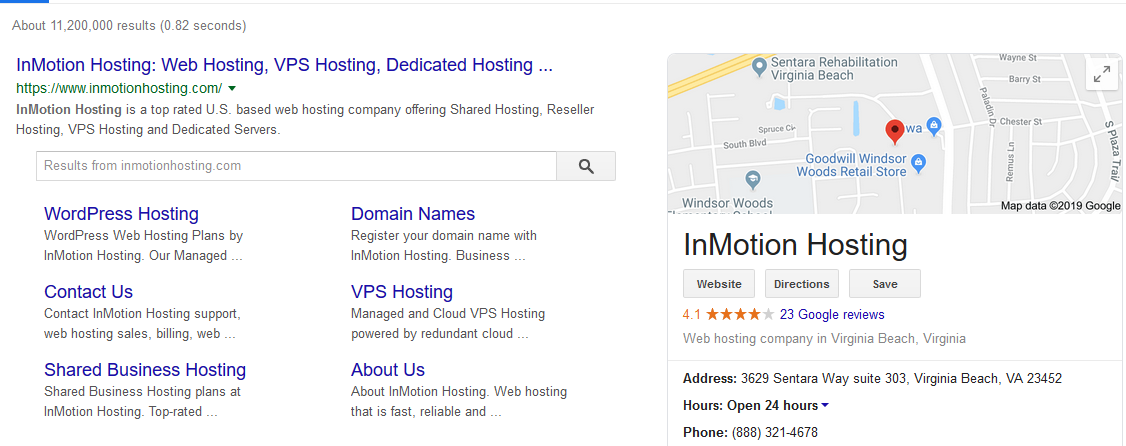The image depicts a Google search results page indicating approximately 11,200,000 results returned in 0.82 seconds. The prominent result highlights "InMotion Hosting" with its website URL, www.inmotionhosting.com, and describes it as a leading U.S.-based web hosting company. InMotion Hosting offers a variety of services including shared hosting, reseller hosting, VPS hosting, and dedicated servers. Below this introduction, there is a box labeled "Results from InMotionHosting.com". The detailed list within this box includes:

1. **WordPress Hosting**: Dedicated WordPress web hosting plans by InMotion Hosting.
2. **Contact Us**: Information on contacting InMotion Hosting support for web hosting sales, billing, and other queries.
3. **Shared Business Hosting**: Shared business hosting plans offered by InMotion Hosting, which are highly rated.
4. **Domain Names**: Services for registering domain names with InMotion Hosting.
5. **VPS Hosting**: Managed and cloud VPS hosting powered by RedundantCloud.

The page emphasizes InMotion Hosting's comprehensive web hosting solutions tailored for various needs.